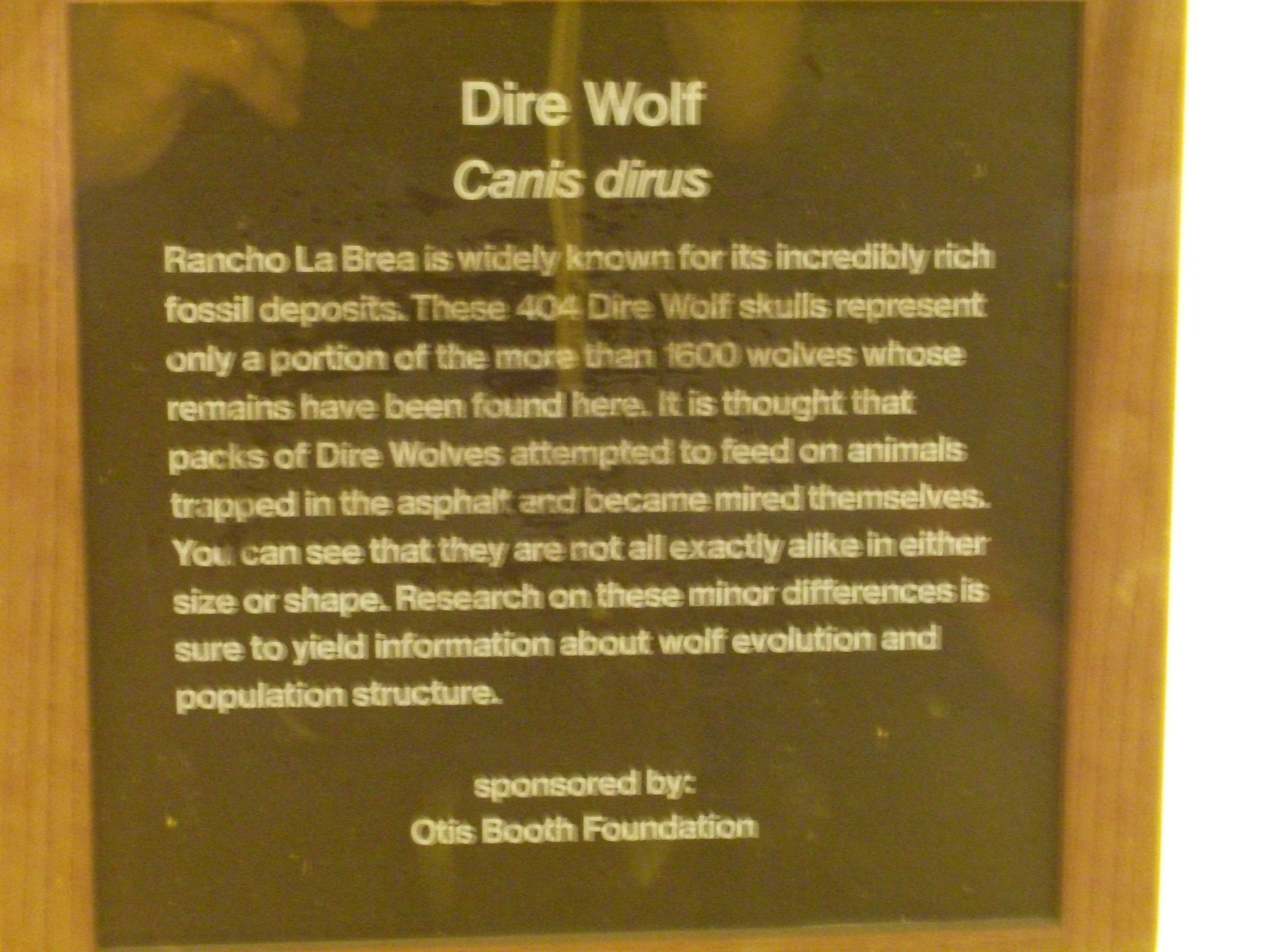The image depicts a very blurry photograph of an informational placard, likely taken in a museum. The placard is enclosed in a brown wood grain frame and covered by a highly reflective piece of glass or plastic. The top left corner of the image shows a reflection of a person holding a camera. The placard itself features a black background with large, bold white text at the top reading "Dire Wolf" and "Canis Dirus." Beneath this, there is a column of much smaller white text. The text notes that "Rancho La Brea is widely known for its incredibly rich fossil deposits. These 404 dire wolf skulls represent only a portion of the more than 1,600 wolves whose remains have been found here. It is thought that packs of dire wolves attempted to feed on animals trapped in the asphalt and became mired themselves. You can see that they are not all exactly alike in either size or shape. Research on these minor differences is sure to yield information about wolf evolution and population structure." The content is sponsored by the Otis Booth Foundation.